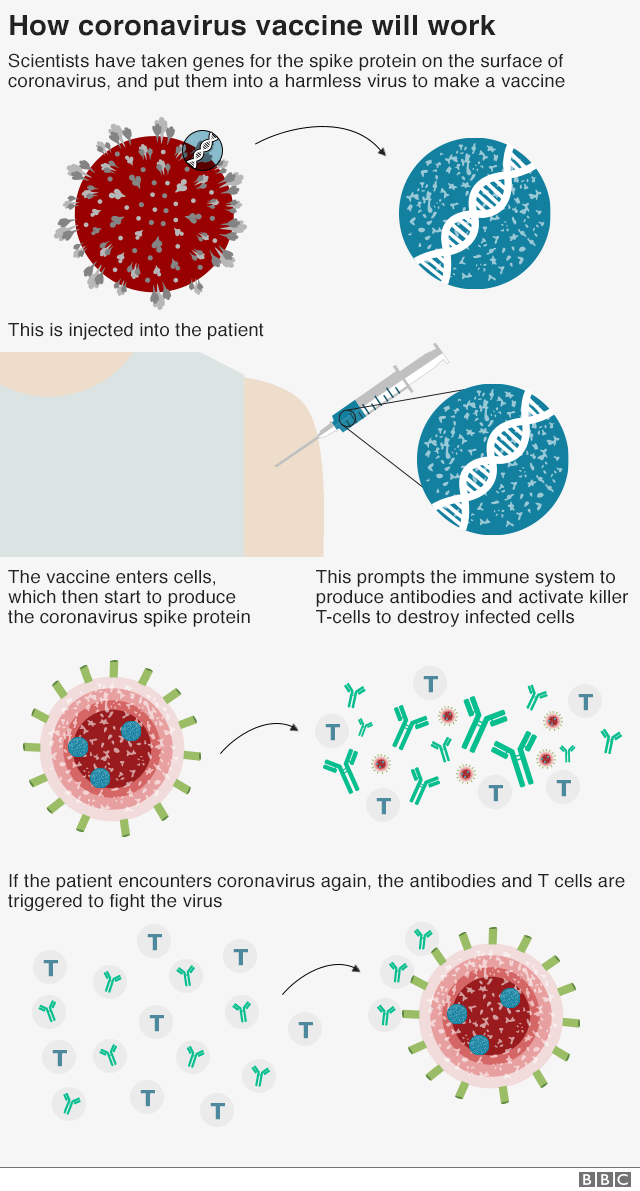The image is an informative poster titled "How the Coronavirus Vaccine Works." At the top, the poster explains that scientists have engineered a vaccine by inserting genes for the COVID-19 spike protein into a harmless virus. The visual elements include a red circle representing the coronavirus with spike proteins, connected by an arrow to a blue circle depicting the DNA strand. 

The poster goes on to illustrate the vaccination process: a needle injecting the DNA strand into a patient's arm. The diagram highlights that once inside the body, the vaccine enters cells and prompts them to produce the spike protein. This process activates the immune system, leading to the creation of antibodies and the activation of killer T-cells, which target and destroy infected cells.

Further down, the poster shows an illustration of a cell infected with the virus alongside activated T-cells. This visual signifies the immune response if the patient encounters the coronavirus again, with antibodies and T-cells ready to combat the virus. 

Overall, the poster provides a detailed explanation and visual representation of how the coronavirus vaccine generates an immune response to protect against future infections.